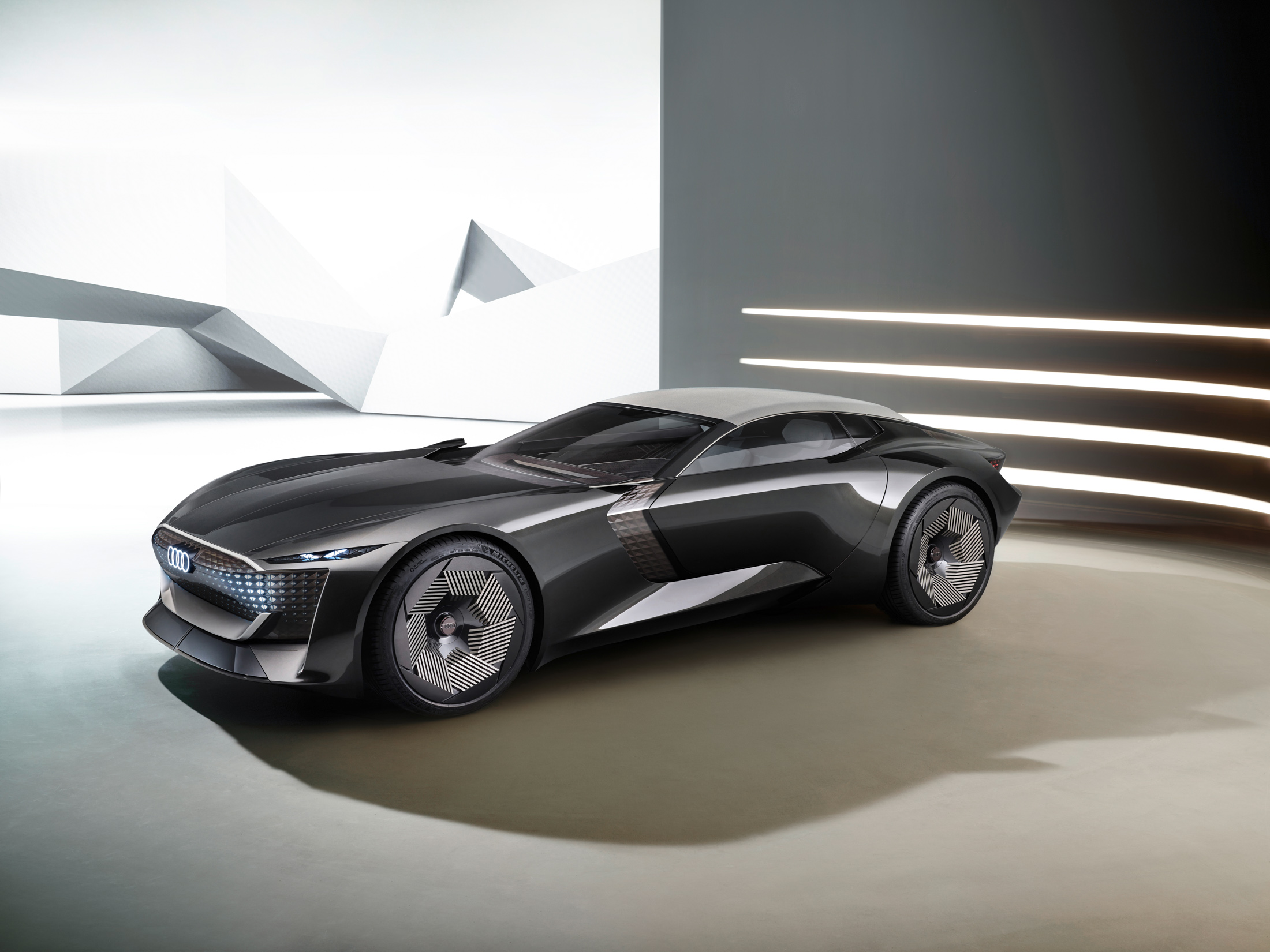The image showcases a highly detailed, digitally rendered sports car in a landscape orientation, resembling a scene from a video game. The sleek vehicle, which appears to be an Audi, features a low-profile design with a distinct Audi logo on its solid, screen-like grille. The car's body is a dark charcoal color with a light gray roof and narrow headlights that accentuate its modern aesthetic. The innovative, large silver wheels are set flush within the wheel wells, further enhancing its streamlined appearance. The car is positioned in a sophisticated display environment, characterized by angular, textured walls and a light-colored, horizontally striped backdrop, with an off-white floor, underscoring the car's futuristic vibe and potential for groundbreaking innovation.